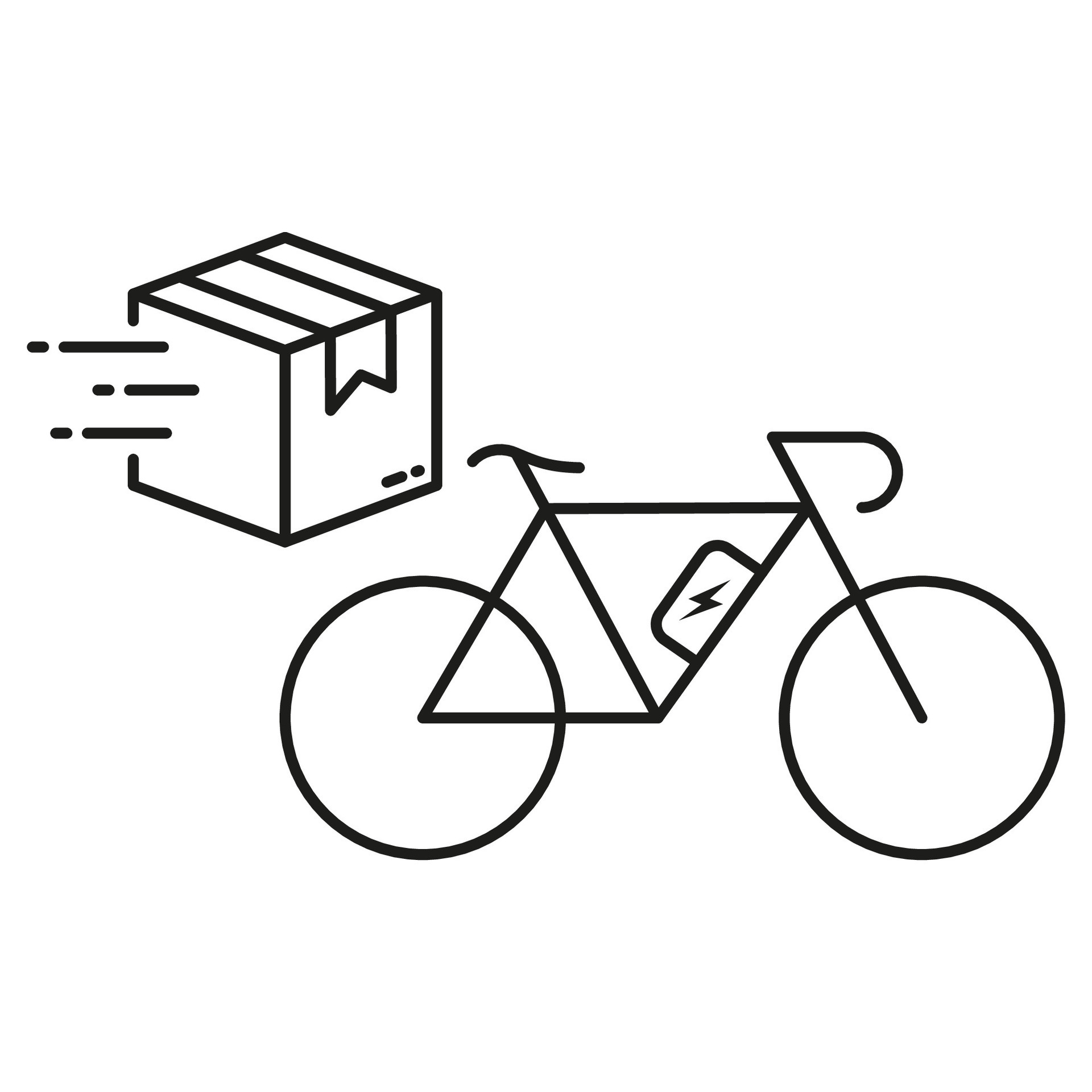The image is a black and white vector illustration set against a white background, featuring two distinct yet related elements: a bicycle and a package. To the left, there is a small, cubic cardboard box with an indication of motion conveyed by three horizontal lines extending from its left side, suggesting it is moving swiftly. The box also has a line on top resembling tape sealing it shut. To the right, there is a detailed drawing of a racing-style bicycle, characterized by its curved handlebars. The bicycle includes two large circular wheels and, notably, a small rectangular box with a lightning bolt symbol mounted along the frame, implying it is an electric bike. The deliberate placement and design of both the package and the bicycle suggest the theme of fast delivery, possibly indicating a speedy delivery service facilitated by the electric bike.